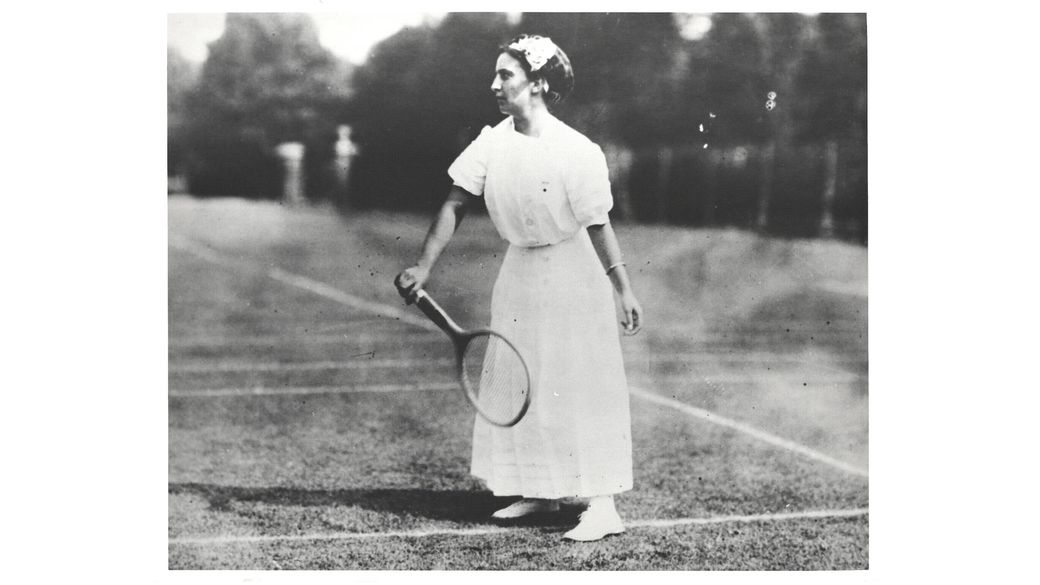This black-and-white, grainy photograph depicts a woman on an old-fashioned tennis court. She stands in the center, posed with a wooden tennis racket in her right hand, facing left in a preparatory stance. The tennis court, characterized by white painted lines, appears to be made of grass. The image’s background is blurred with an indistinct tree line and a fence, giving a sense of depth and age to the scene.

The woman is wearing a cinched white dress with short sleeves down to her elbows, complemented by a bracelet and white shoes, possibly tennis footwear. She has her hair pulled back with what seems to be a light hat or head wrap, possibly adorned with a butterfly decoration. Her shadow extends to the left, indicating the sun is positioned behind her at an angle. The overall texture of the photo is heavily grainy, adding to its antique charm, and the aged appearance of the image makes it seem almost foggy.